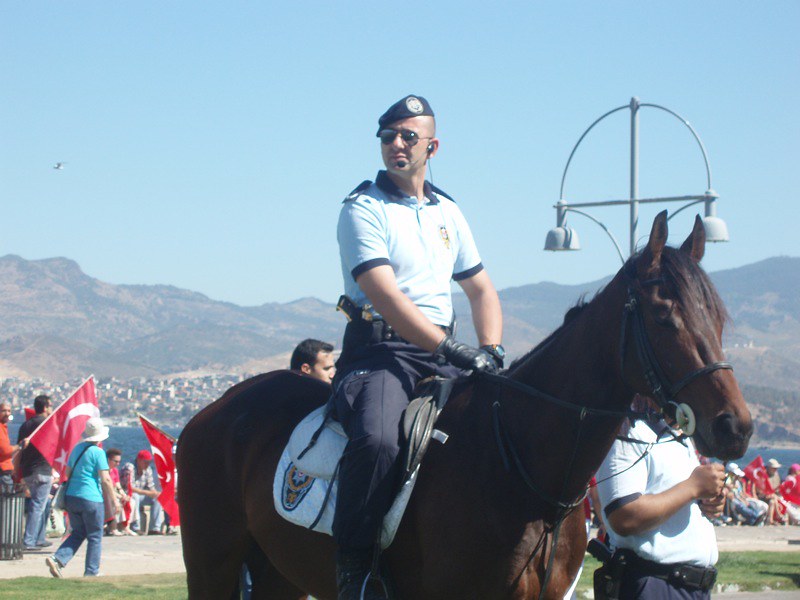The photograph captures a detailed scene featuring a mounted police officer on a striking brown horse during a public event. The officer, with minimal hair or bald, is seen wearing sunglasses, black gloves, and a black beret-like hat. Equipped with a white short-sleeved polo shirt featuring black cuffs and a black collar, the officer also sports a microphone headset extending from his ear to his mouth, and a visible security emblem on his saddle. He is seated calmly on his horse, which is positioned with its head facing right and its rear to the left. 

The background reveals a picturesque landscape with hills and a body of water, possibly a river, alongside a residential area nestled in the hills and distant mountains under a clear blue sky. The scene is bustling with numerous people, indicative of a significant gathering or event. The crowd, many dressed in red and holding flags adorned with a crescent and star, seems animated yet orderly. A dirt path can be spotted along with a garbage can in the lower left corner, hinting at a public area. Another person, donning a similar uniform and carrying a gun in a holster, is standing near the horse, complementing the overall sense of security and surveillance presented in the image.